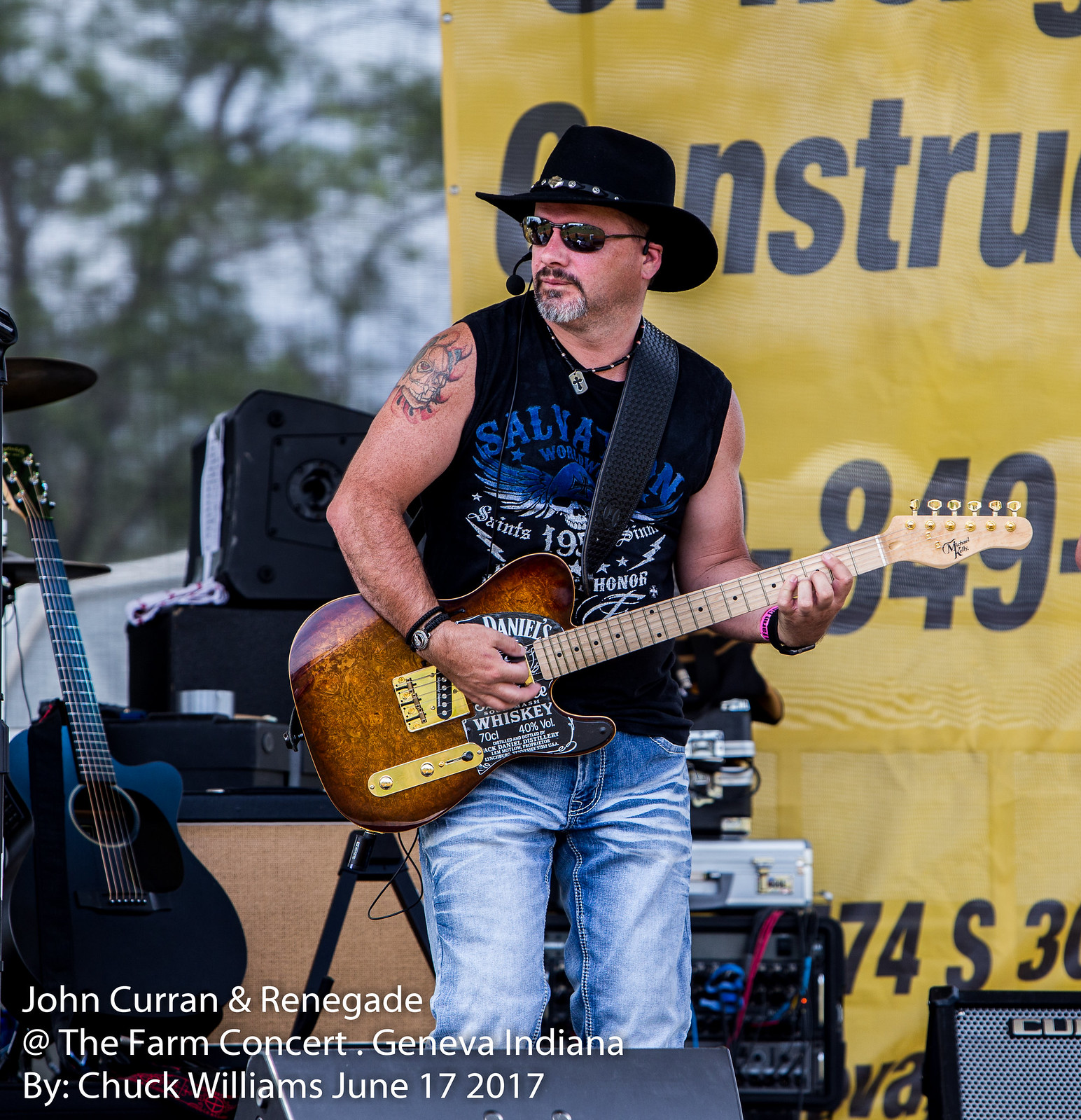The image features a man on stage playing a marbled brown electric guitar adorned with a Jack Daniels whiskey logo. He wears black sunglasses and a black cowboy hat, complementing his black sleeveless tank top emblazoned with partially obscured lettering that includes "Salvation" and "Saints and Sinners." The man's visible tattoo on his upper right arm depicts a creature, possibly a dragon, with red flames around it. The guitar's strap is thick, black, and likely leather, cutting through part of the shirt's text. In front of him sits an amplifier and a few speakers among various audio equipment. Behind him, a yellow sign is mostly obscured. On the lower left of the image, a sleek, shiny black acoustic guitar rests on a stand, and part of a drum set is visible in the background. The text at the bottom left of the image reads, "John Crew and Renegade at the Farm Concert Geneva, Indiana by Chuck Williams, June 17, 2017."